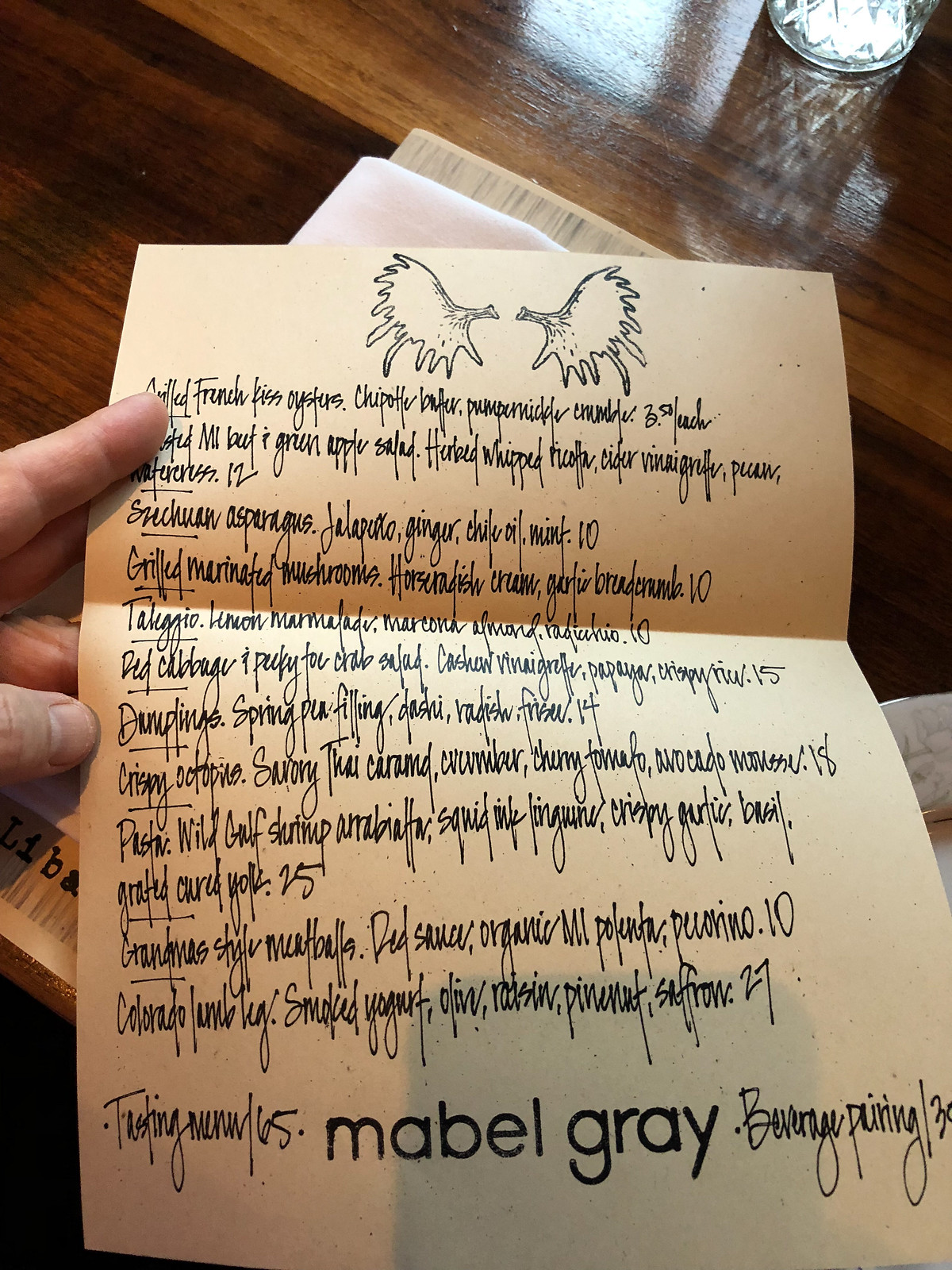Photographed from the left side of the frame, a hand extends holding a piece of paper. The hand, belonging to an unseen individual, is positioned such that only the thumb and one finger are visible. The paper held between the digits displays a handwritten menu in elegant script. At the top of the menu, an illustration resembling antlers or horns is distinctly visible, adding a unique decorative touch.

The menu features a variety of tantalizing items, though some details are partially obscured:

1. Grilled French kiss oysters with chipotle and possibly pepperidge, priced at $3.50 each.
2. [Indistinct] grown apple salad with whipped ingredients, fresh cider vinaigrette, pecans, and watercress, listed at $12.
3. Szechuan asparagus with ginger, chili oil, and mint, priced at $10.
4. Grilled marinated mushrooms accompanied by horseradish cream, garlic bread, and [indistinct], for $10.
5. [Indistinct] lemon marmalade, marcona almonds, and srirachino, also at $10.
6. Red cabbage and [indistinct] crab salad, priced at $15.
7. Dumplings with a spring [indistinct] filling, radish, and [indistinct], for $14.
8. Crispy [indistinct], ending the list.

At the bottom of the menu, 'Mabel Gray' is inscribed, presumably indicating the name of the establishment. The detailed descriptions and artistic flourishes suggest a unique and upscale dining experience.